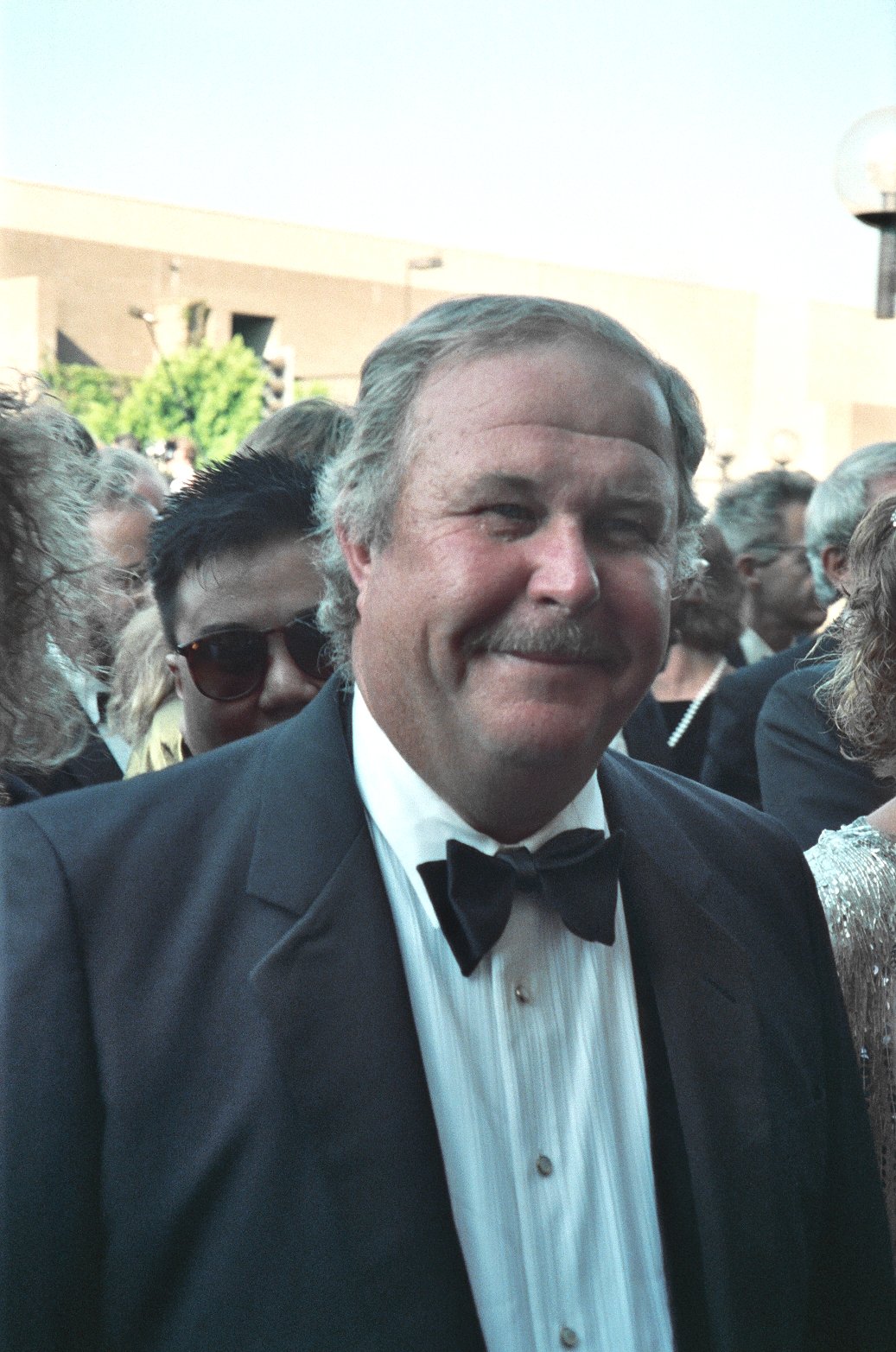This image prominently features the late American actor Ned Beatty, dressed in a black tuxedo suit with a white button-up shirt adorned with silver buttons, and a black bow tie. Ned, an older gentleman likely in his 60s, is smiling and looking off-camera. His hair and mustache are grey. Behind him, a man with spiky hair and dark sunglasses looks towards the camera, positioned just over Ned's shoulder. Additionally, part of a woman in a shiny dress with short brown hair can be seen beside Ned. The background shows a crowd of people, all dressed in suits, enhancing the formal atmosphere. The setting appears to be outside, with green leaves and a building visible in the top left corner, along with the sky.